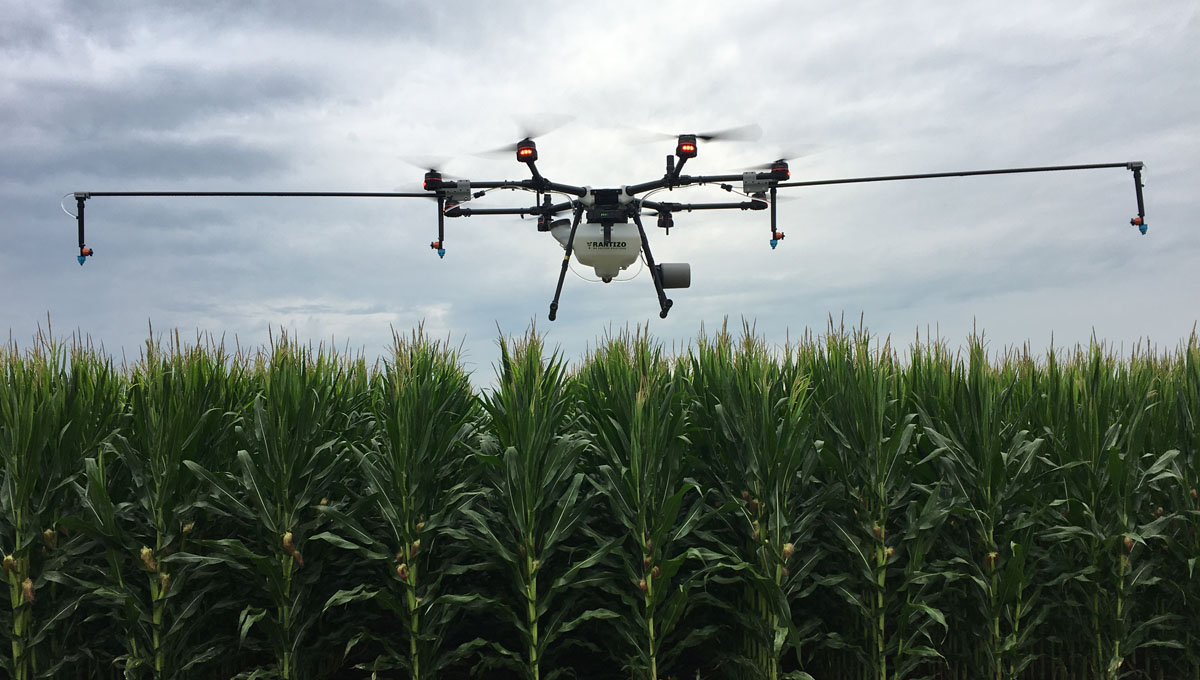The photograph depicts a large drone hovering over a dense field of tall, healthy green corn crops on an overcast day. The drone is equipped with six propellers arranged in a star-shaped pattern that keep it airborne. Attached to the drone's white body, which features the branding "Rentizo" in black text, are long black arms extending from the sides. These arms have tubing connected to them, which ends in nozzles for dispensing protective chemicals, water, or fertilizer. The drone also features a tank underneath for storing these substances. Additionally, there are two orange-colored lights spaced about two feet apart, positioned near the back propellers. The cloudy sky provides a muted background, emphasizing the lushness of the cornfield below.